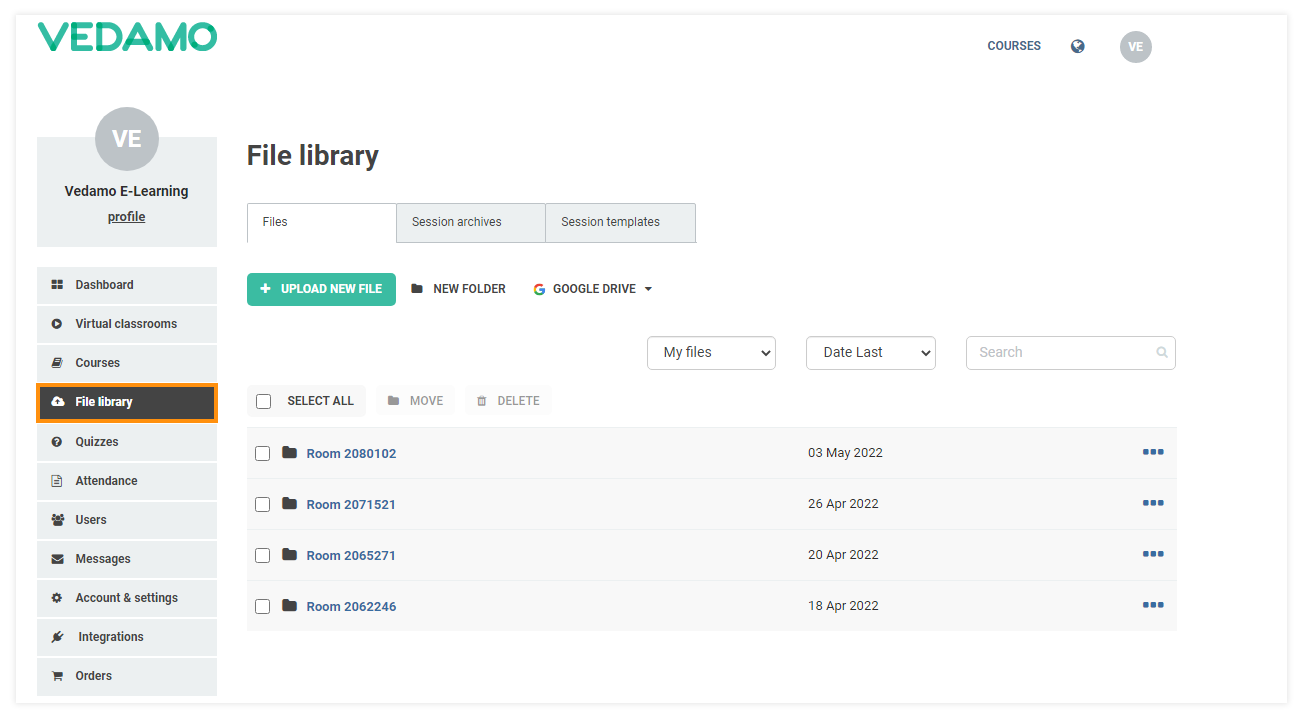The image showcases a detailed interface of an e-learning platform with a white background. The entire layout is outlined with light blue lines. In the top left corner, the word "VEDAMO" appears in green letters. Adjacent to it on the right is the word "courses" accompanied by a tiny green circle. Further to the right, there's a gray circle containing the letters "VC".

On the left side of the image, a blue box is visible, inside which is a circle with "VE" inscribed in it, followed by the text "VEDAMO e-learning profile". Below this, there are several smaller blue boxes containing various options: "Dashboard", "Virtual Classrooms", "Courses", a highlighted "File Library" in red, "Quizzes", "Attendance", "Users", "Messages", "Account and Settings", "Integration", and "Orders".

To the right, the "File Library" section is displayed prominently. This section includes tabs labeled "File Tab", "Session Archives", and "Session Templates" in blue. There are options to "Upload New File" in green, create a "New Folder in Google Drive" marked by Google's signature red, yellow, green, and blue "G", as well as "Select All" with a corresponding checkbox, and buttons for "Move" and "Delete".

At the top, three boxes are shown: "My Files" with a dropdown menu, "Date List" with another dropdown menu, and a "Search" box. Below these, four titles are displayed, each preceded by a checkbox. These titles are associated with room numbers and corresponding dates: "Room 3" dated "03rd of May 2022" with three blue dots, "Room 26" dated "26th of April 2022" with three blue dots, "Room 20" dated "20th of April 2022" with three blue dots, and "Room 18" dated "18th of April 2022" with three blue dots.